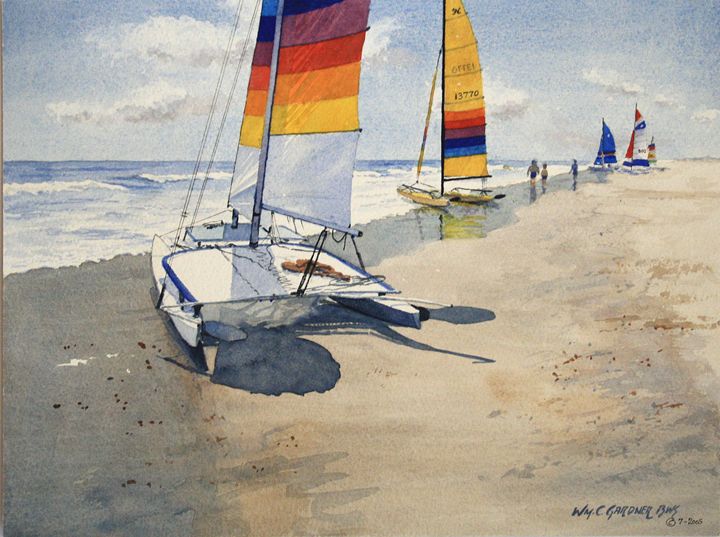A detailed painting of a seashore features several modern sailboats resting on a light brown sandy beach with splotches of mid-brown and gray. The sand lightens to almost gray where waves have wet it near the boats, indicating high tide. The dark blue ocean extends to the left, gradually changing to foamy white waves as they crash onto the shore. The dark blue sky lightens towards the horizon and the right side, filled with fluffy clouds that gather in the center and right.

In the foreground, a white sailboat with a multicolored, striped sail—featuring light blue, dark blue, maroon, orangish red, orange, yellow, and prominent white stripes—stands out. This sailboat also has black wiring stretching towards the sail. Next to it, another sailboat boasts a bright yellow hull and mostly yellow sail adorned with the number 13770 in black, surrounded by a frame of stripes in orange, red, purple, dark blue, light blue, and yellow, with yellow wiring.

Three individuals are near the water's edge, positioned to the right of the yellow sailboat. Nearby, there are three other boats: one with a large dark blue sail, another with a mainly white sail accented by a blue stripe and a red tip, and a final boat which is difficult to discern in detail. The artist has signed the painting in the lower-left corner, although the signature is hard to read. The scene is likely captured during daylight, suggested by the light and the presence of people.